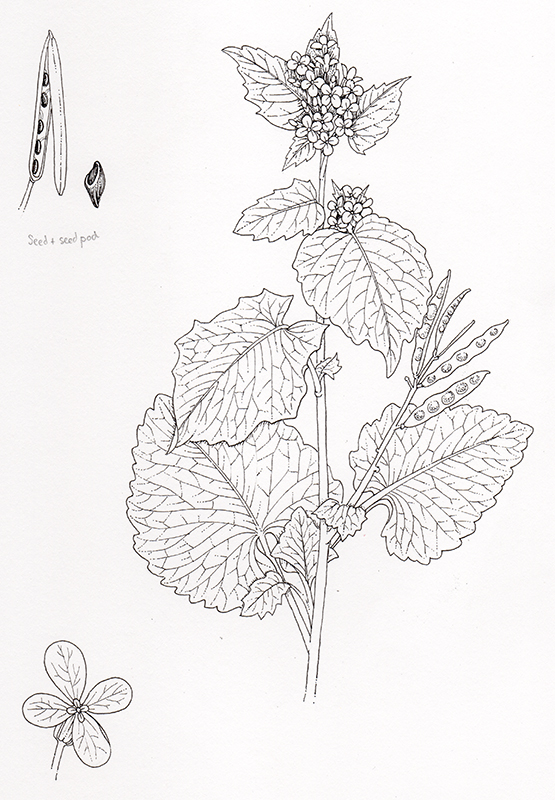The image is an intricate black-and-white drawing of a botanical subject. At the center of the image is a long-stalked plant adorned with numerous broad leaves. At the top of the plant, a detailed flower blooms, composed of four distinct petals. Attached to this flower are various seed pods, resembling peapods, each containing five pointy seeds that have a curved, beak-like appearance. The flower itself is depicted with detailed veins running through its petals. On the lower left-hand corner of the image, there is a close-up view that highlights the flower and its intricate vein patterns further. The entire image has a freehand-drawn look, created using black pencil or ink on a white background, giving it a sketch-like quality typical of botanical illustrations found in vintage books. The drawing is labeled with 'seed' and 'seed pod' annotations, emphasizing the educational purpose of showcasing the plant's reproductive elements.